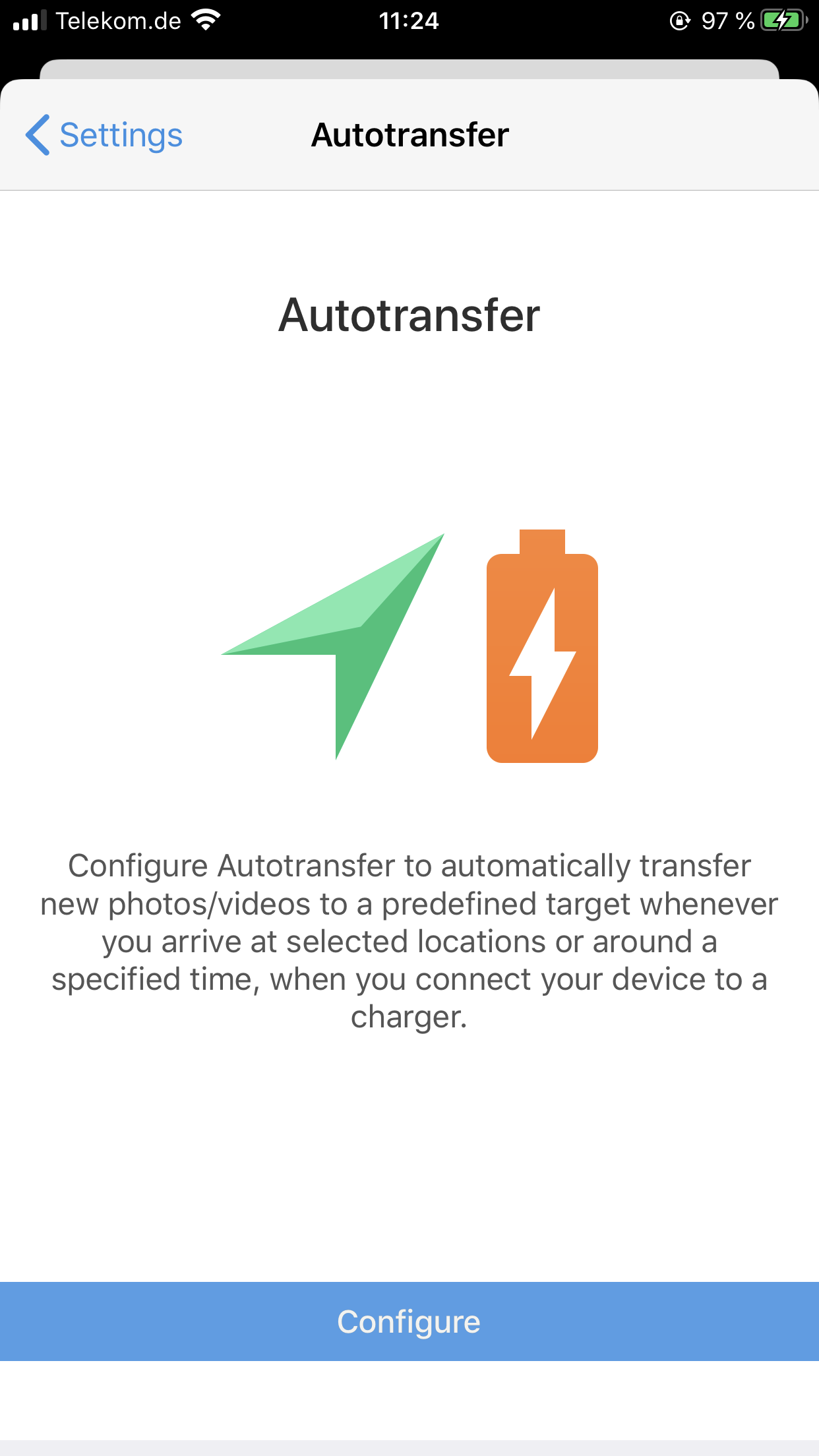Screenshot of the interface for the "Auto Transfer" settings page in portrait mode:

- **Status Bar**: 
  - Top left corner: "Telecom Point DE"
  - Top center: Time stamp "11:24"
  - Top right corner: Battery indicator at 97%

- **Interface Details**:
  - Below the status bar: A blue back button labeled “Settings”
  - Page title in black text: "Auto Transfer"
  - Background: Predominantly white

- **Visual Elements**:
  - A large, green gem-like arrow pointing towards the upper right corner
  - An orange battery icon with a lightning bolt symbol in the center

- **Instructional Text**:
  - "Configure auto transfer to automatically transfer new photos and videos to a predefined target whenever you arrive at selected locations or around a specified time when you connect your device to a charger."

- **Action Button**:
  - A blue button labeled “Configure”

**Interpretation**:
This page allows users to set up automatic transfers of their photos and videos to a designated storage service, such as Amazon or Google Drive, ensuring their media is regularly backed up without manual uploads. The transfers can be triggered by connecting the device to a charger at specific times or when arriving at selected locations.